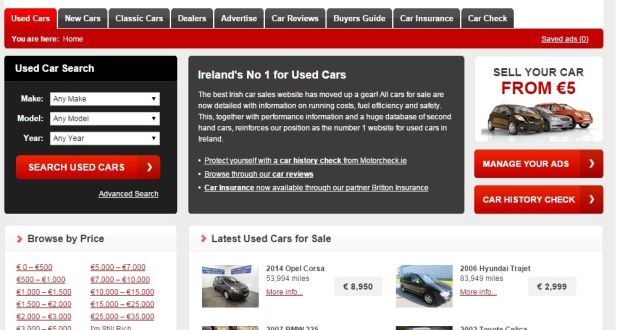The image depicts a meticulously designed web page from an Irish car sales website, specializing in used cars. The visually dominant theme incorporates a sleek color palette of white, black, and red, with text presented in these contrasting colors for clear readability. 

At the top of the page, a navigation bar features tabs including "Used Cars" (highlighted in red to signify its current selection), "New Cars," "Classic Cars," "Dealers," "Advertise," "Car Reviews," "Buyer's Guide," "Car Insurance," and "Car Check." Beneath the navigation bar, a breadcrumb trail indicates the user's current location within the site: "You are here: Home."

A prominent search box labeled "Used Car Search" allows users to filter vehicles by "Make," "Model," and "Year," with a bold red "Search Used Car" button ready for activation. To the right of the search functionality, a banner proudly proclaims the site's status as "Ireland's number one for used cars." It boasts about enhanced features detailing running costs, fuel efficiency, safety metrics, and performance information, all contributing to the website's repute as the premier destination for secondhand car purchases in Ireland.

Further down, the site’s offerings are segmented into sections such as "Protect Your Car," "Browse Car Reviews," and "Car Insurance available." Displayed below these - an assortment of car prices and a scrolling list labeled "Latest Used Cars for Sale," featuring images and details of available vehicles like a 2014 Opel Corsa and a 2006 Honda Trajet.

The detailed layout and comprehensive information provide a user-friendly experience for potential car buyers.